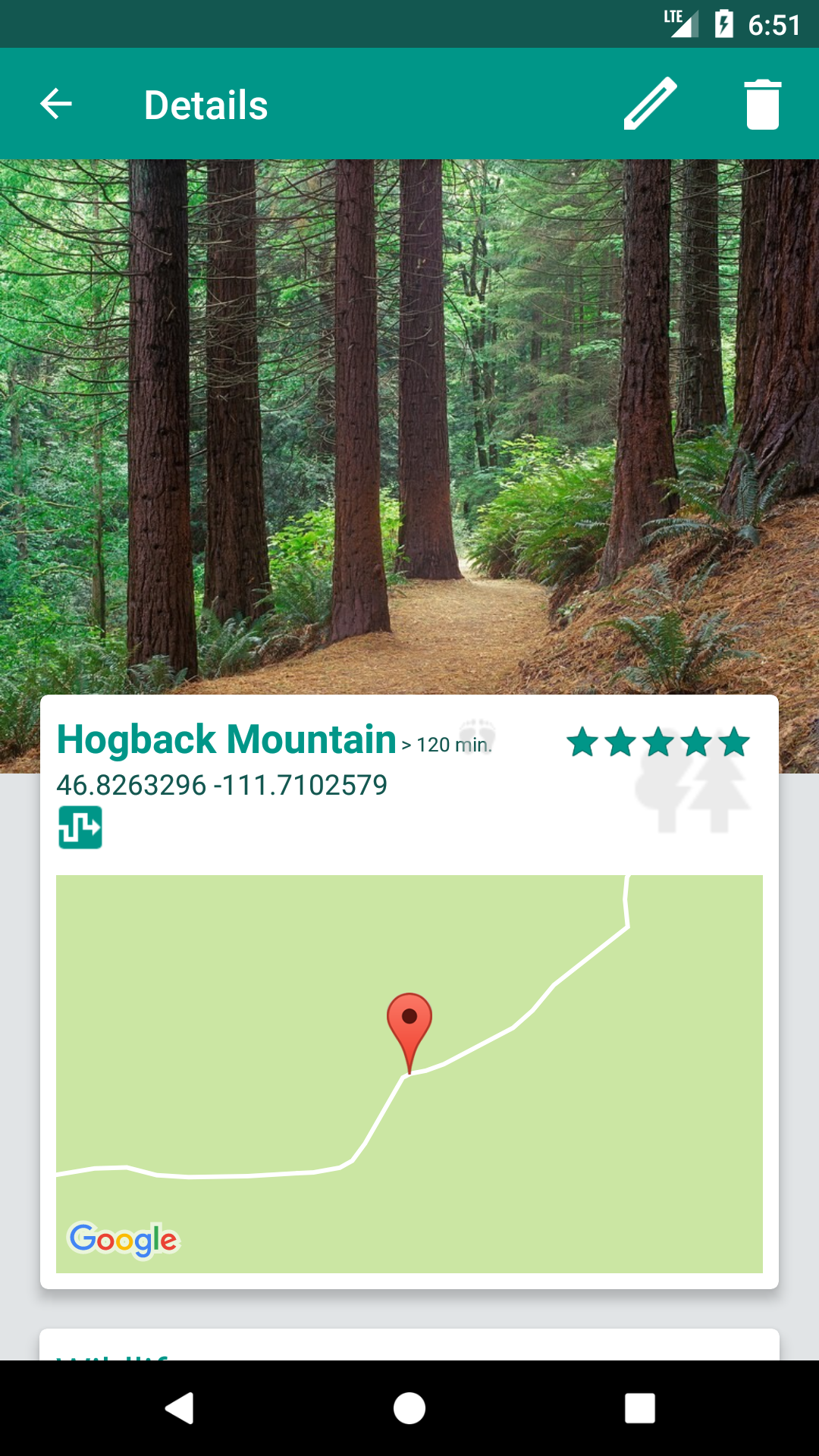This image is a screenshot of a mobile web page or application. At the very top of the screen, there's a dark green status bar displaying "LTE" on the right, alongside a signal strength icon with four bars, an icon of a computer, a charging battery symbol, and the time reading 6:51. The battery icon indicates that the phone is currently charging.

Below the status bar is a lighter green header section that contains the title "Details" with a left-pointing arrow beside it. To the right of this title, there are icons of a pencil and a trash can.

Under the header is a picturesque photograph depicting a serene mountainscape. The image showcases a trail winding through light brown dirt, surrounded by ferns and tall trees, embodying a tranquil mountain setting.

Beneath the photograph, there is a large square map highlighting the location "Hogback Mountain," which is noted to be 120 minutes away. The map area is rated five stars and includes precise GPS coordinates: 46.8263296, -111.7102579. The map itself features a single road snaking through its center, which has a red marker indicating the specific spot of Hogback Mountain. In the bottom left corner of the map, the word "Google" is visible, signifying the map's source.

Finally, at the very bottom of the screen, there is a black bar containing three navigation icons: a triangle, a circle, and a square, most likely representing the phone’s basic navigation buttons.